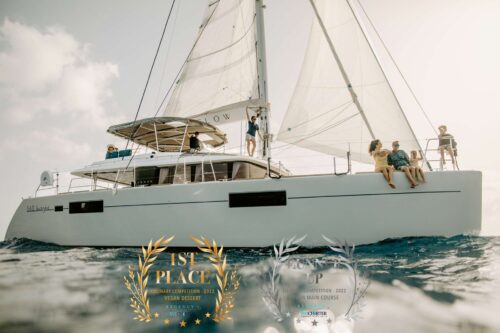This image features a large white yacht sailing on the ocean under a somewhat cloudy sky. The vessel, shaped in a rectangular form, includes a base and a covered area likely for the captain. Prominently, there are two sails: a larger one on the left and a smaller, looser sail on the right. On deck, a middle-aged couple and a young child, perhaps around five years old, are seated together, suggesting a family. An older woman sits on a chair nearby, engaging in conversation with them. Additionally, a woman dressed in a blue shirt and skirt stands at the rear of the yacht. Another individual is seen standing on the roof of the cabin, leaning against the mast. The water in the lower third of the picture has a blue tinge. In the foreground, there are two award stamps: one is a gold wreath denoting first place, and the other, silver, both partially obscured and unreadable.